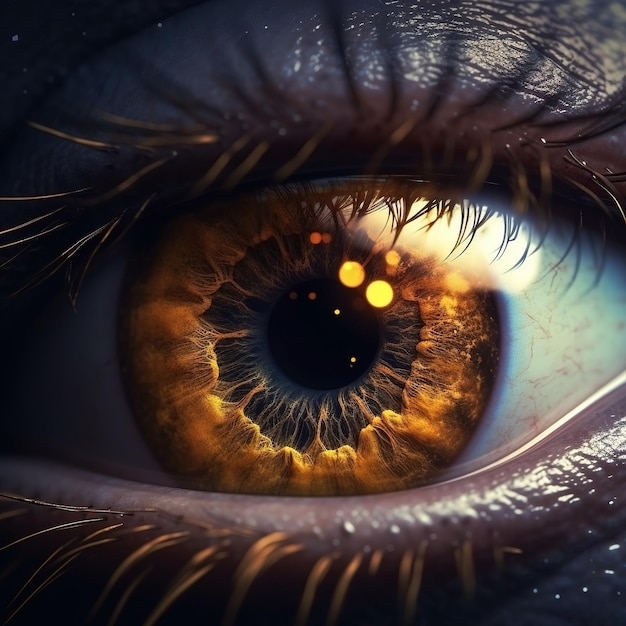The image is a very detailed and clear close-up of an eye, showcasing its intricate features with natural brightness. The eye, possibly a hazel or golden light brown color, is centrally positioned and open, looking directly at the camera. The pupil is black and surrounded by orbs of yellow and brown, with a pinpoint black center. You can see a distinct contrast between the white part of the eye and the colorful iris. Luscious eyelashes frame the eye, visible both at the top and bottom of the image. The surrounding skin appears smooth. The photograph is devoid of any text or numbers, focusing entirely on the eye's natural beauty.